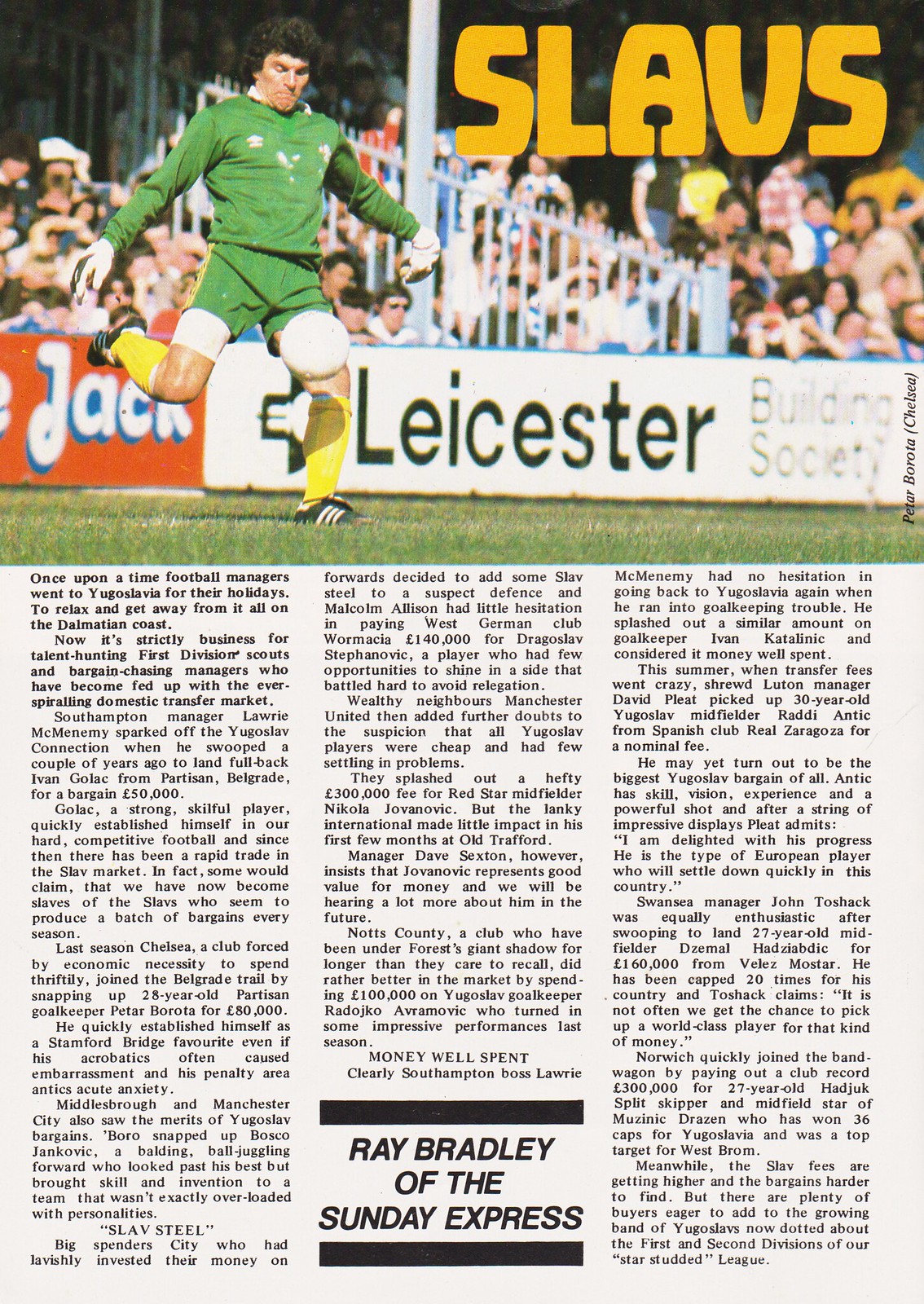This image is a page from a sports program or magazine, presenting an in-depth focus on football. At the top of the page, there's a headline in bold orange lettering spelling out "SLAVS" with individual yellow letters inside each slab. Dominating the upper half of the page is a vivid photograph of a soccer match featuring a player who seems to be a goalie based on his attire and gloves. This player is donned in a green long-sleeved top, matching green shorts, yellow socks, and Adidas Sambas sneakers. The goalie, who has black curly hair, is captured in the moment of kicking a white soccer ball. Positioned on the playing field with a white and red barricade and a dividing railing visible, the background further showcases the lively crowd in the viewing stands with various advertisements. Among these, a prominent sign reads "LEICESTER BUILDING SOCIETY" and another in white print on a yellow-orange background says "Jack".

The bottom half of the page is filled with numerous paragraphs of small-print text featuring articles and commentary. Notably, there is a highlighted section mentioning Ray Bradley of the Sunday Express. As details emerge from the text, it narrates the transformation within football management, highlighting the Yugoslav influence in scouting and player acquisitions. Various phrases stand out, such as “football managers went to Yugoslavia for their holidays” and “strictly business for talent hunting.” The text underscores the rising demand and value of Yugoslav players in the first and second divisions, alongside the challenges in securing these talents amidst an ever-competitive market. The descriptive nature of the text and its finer details make this page a rich blend of visual and informational content, catering to avid football enthusiasts.